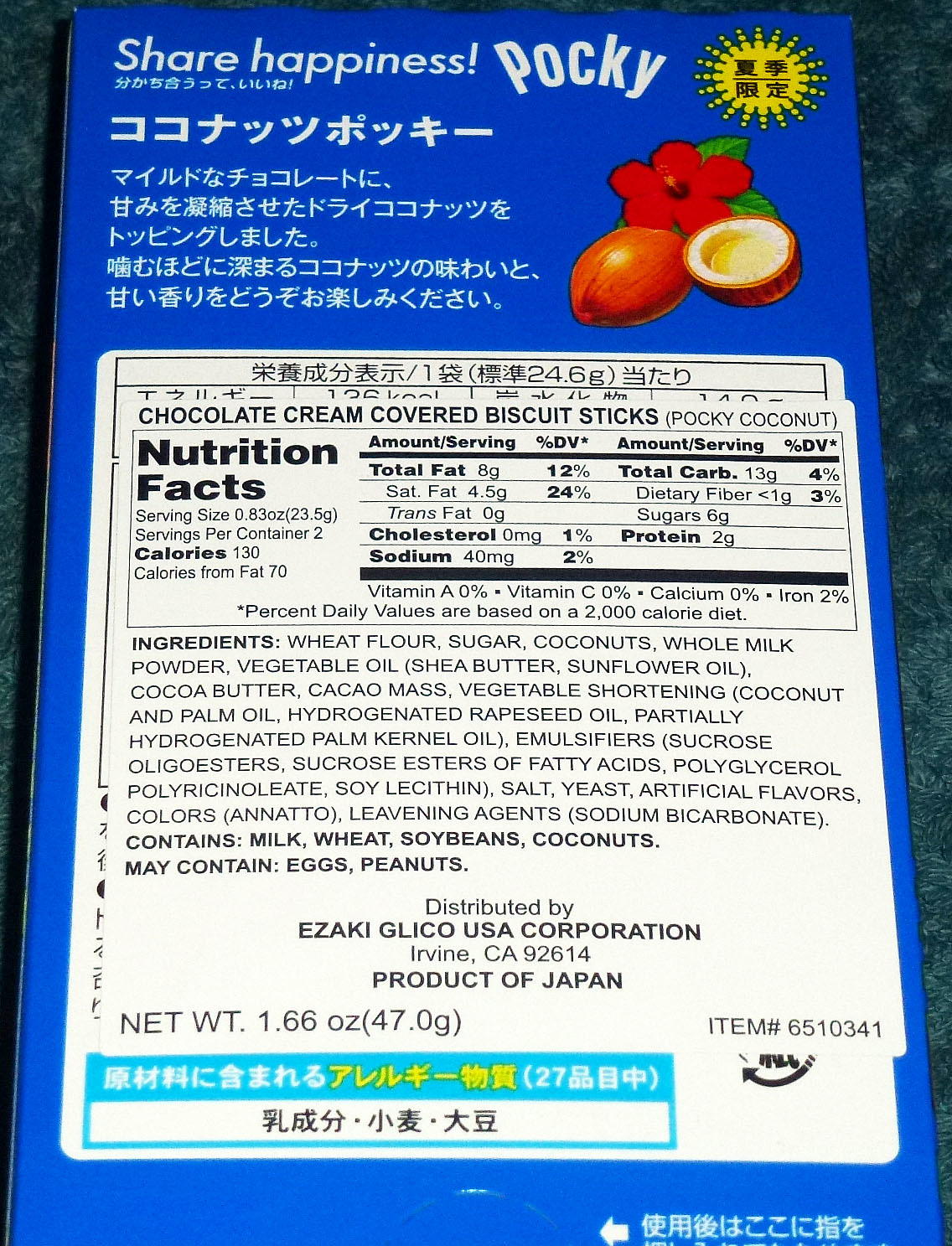The image depicts the backside of a blue container of Pocky Coconut chocolate cream-covered biscuit sticks. At the very top of the container, the words "Share Happiness!" and "Pocky" are prominently displayed in bold white text. To the right of this text, there is a yellow sun-like logo. Below the top section, a series of white Asian-style characters are visible, accompanied by a vibrant red flower with leaves, an orange fruit, and a brown and white object. Beneath these elements, the product name "Chocolate Cream Covered Biscuit Sticks, Pocky Coconut" is clearly printed.

The container also features a detailed Nutrition Facts label outlining various nutritional information. This label includes the nutrient names on the left and their corresponding percentages on the right, with additional vitamin percentages listed below. Following the Nutrition Facts, the ingredients list, distributor details, and location information are provided. At the very bottom, there is a light blue rectangle containing more text, predominantly in white, with some elements in yellow and black.